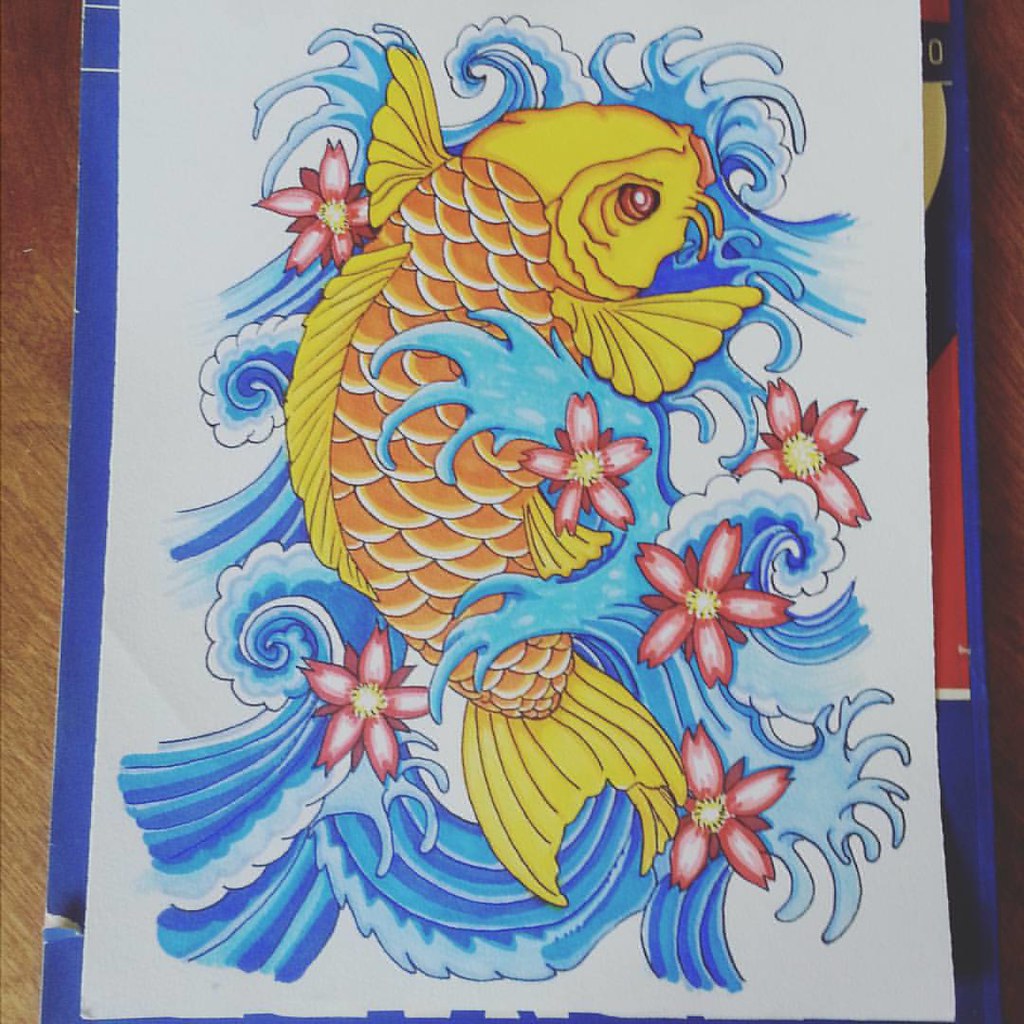The image features a vertically-oriented drawing set against a light brown background, which resembles a tile or stone floor. The drawing rests on a blue-covered book with accents of red, black, and yellow, suggesting it might be a magazine used to stabilize the paper. The off-white sheet of paper showcases a vivid depiction of a koi fish in the center, appearing to leap out of the water. The koi is predominantly gold, yellow, and mustard with hints of orange, featuring red eyes and intricate scales that are oval or semi-circular in shape. Its fins and tail mirror the yellow hue of the rest of its body.

Surrounding the koi are dynamic blue, light blue, and white swirls that evoke the appearance of water and waves. Interspersed among the waves are pink flowers, each with light pink centers that darken to red at the petals' edges. Blossoms with red petals and yellow centers further enrich the scene. The overall composition gives the impression of the fish swimming energetically amidst a flowery aquatic environment.